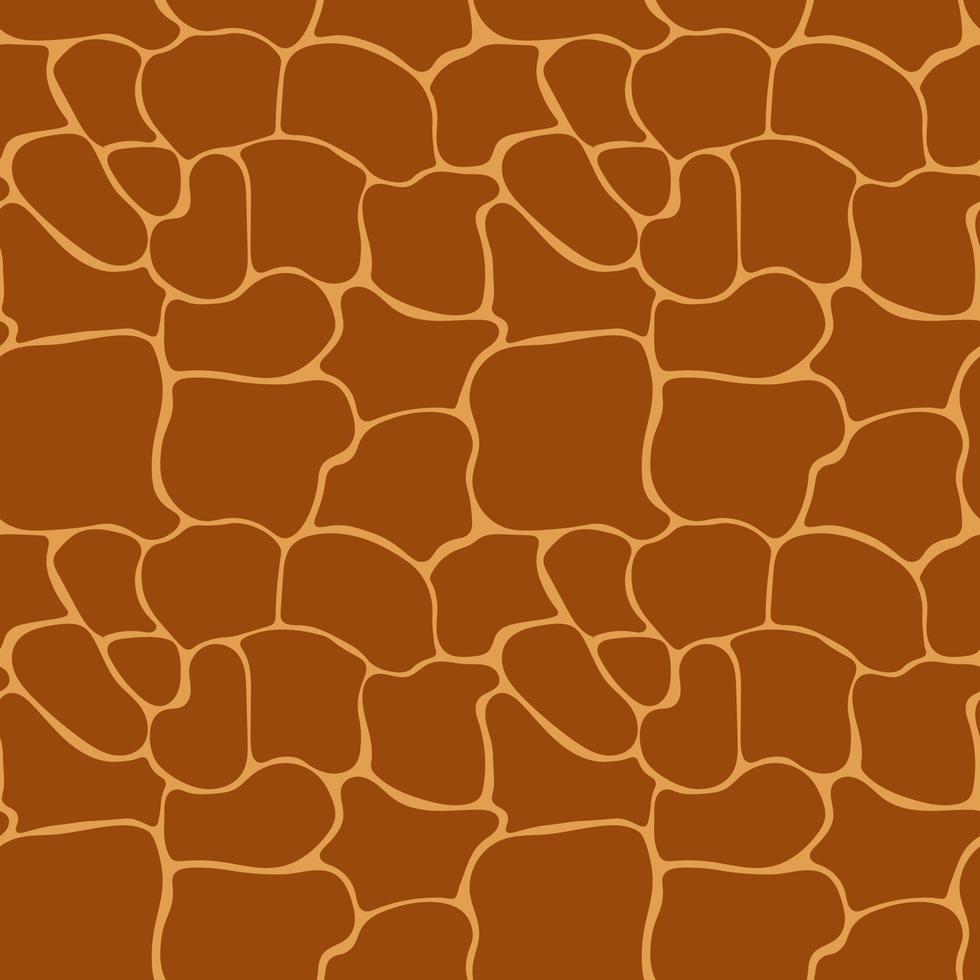The image displays a computer-generated pattern resembling a giraffe print, suitable for backgrounds, borders, or material applications such as book covers, clothing, or wallpaper. The design features an array of irregular and unique shapes in varying sizes, with each shape outlined by a tan or beige color that contrasts against a backdrop of light brown and burnt yellow hues. The shapes, reminiscent of giraffe spots, are densely packed together, creating a cohesive yet intricate and visually intriguing texture.